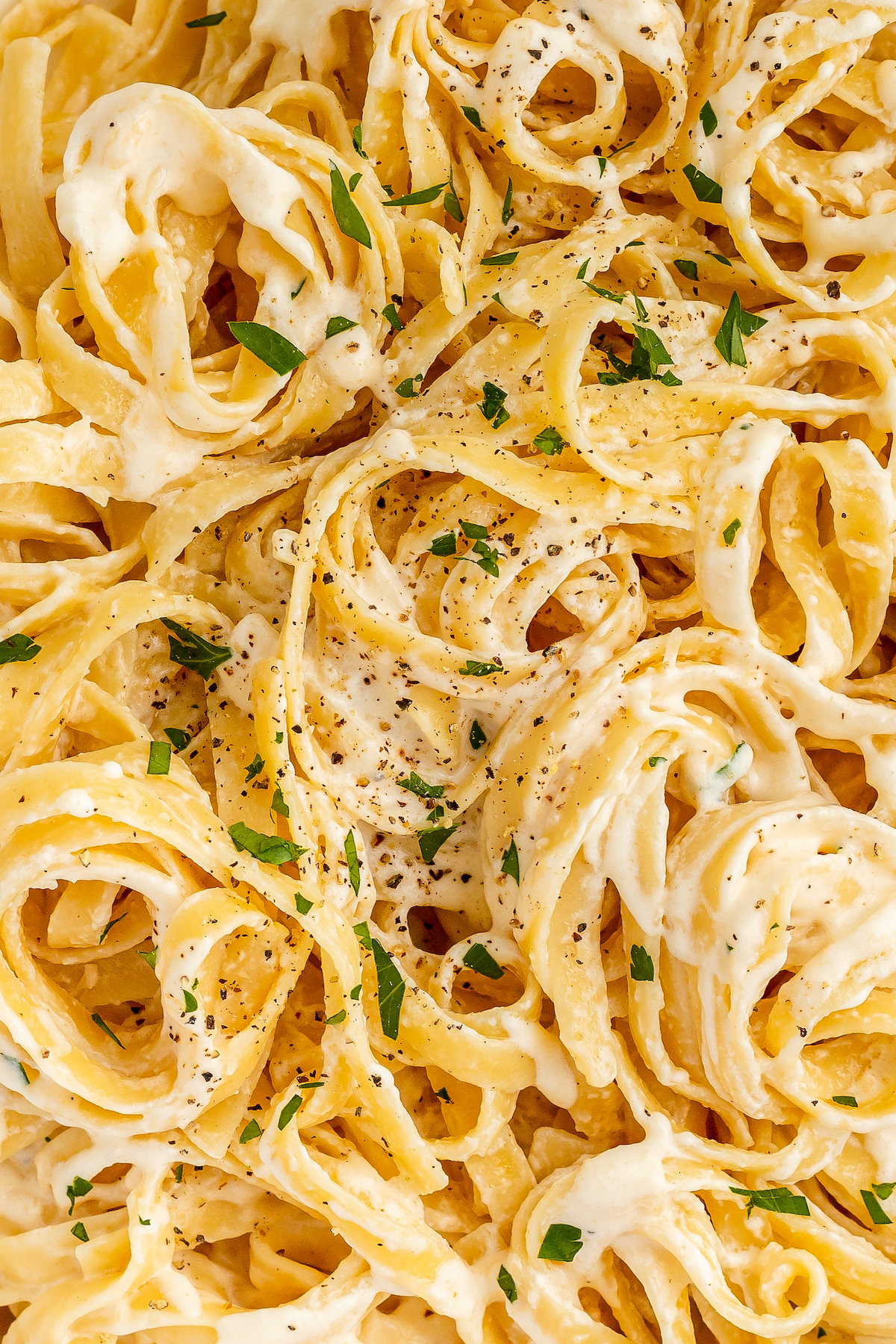This tantalizing and incredibly detailed close-up image showcases a mouth-watering plate of Fettuccine Alfredo. The thin, flat, golden-yellow noodles are tightly swirled and coiled, generously slathered in a thick and creamy white Alfredo sauce. The sauce appears slightly clumpy in places, adding to its rich, indulgent texture. A liberal sprinkling of freshly chopped green herbs, likely parsley or basil, and coarse black pepper flakes adorns the dish, concentrated mainly in the center, creating a vibrant contrast that highlights the earthy green and bold black colors against the creamy white sauce and golden noodles. The tight framing of the photo means that all you can see are the richly coated noodles in their spiraled arrangement, making the creamy pasta the sole focal point of the image. The detailed nature of the photograph emphasizes the textures and colors, capturing the deliciousness of this classic Italian dish.